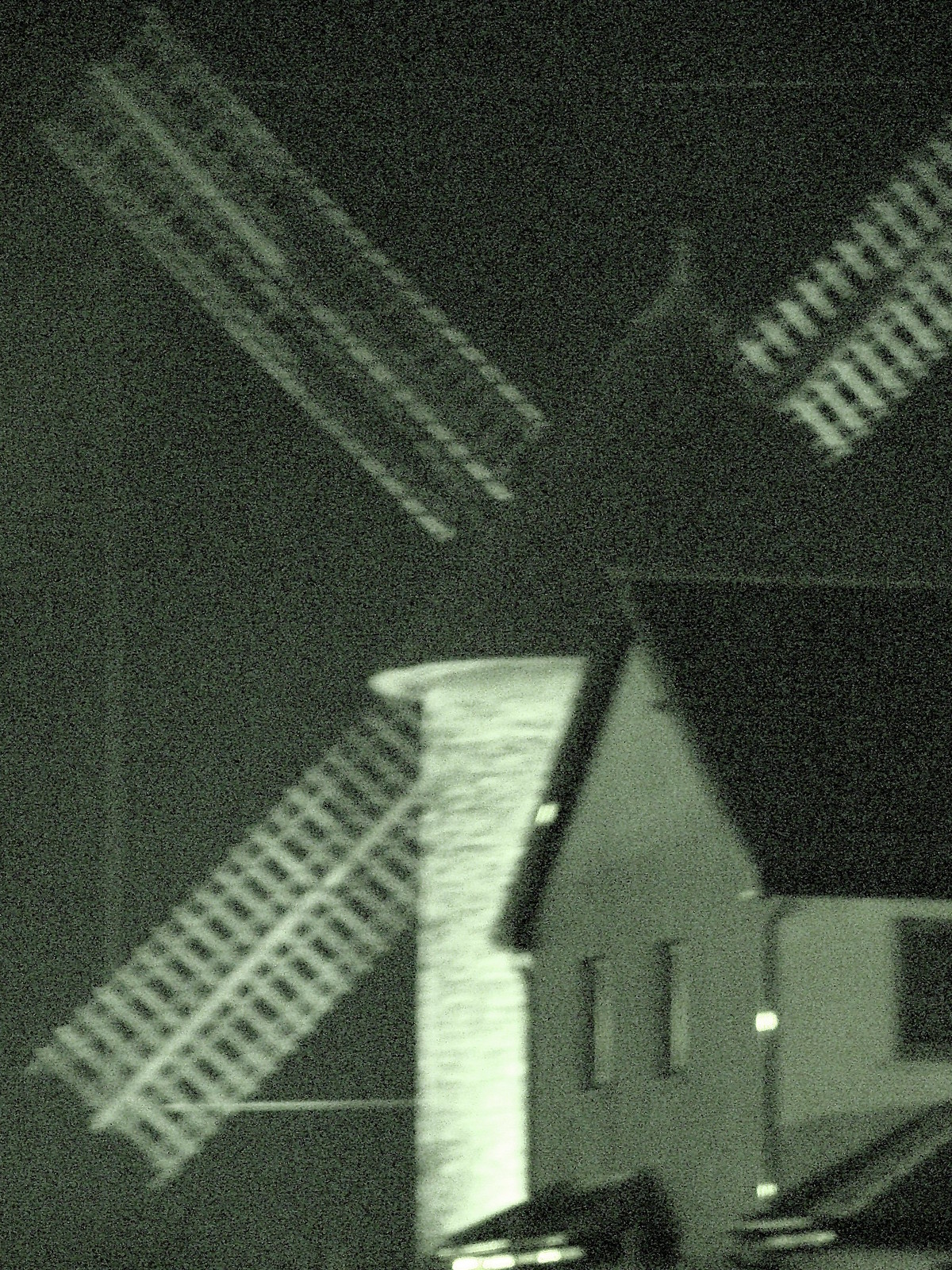This vertically aligned, grainy black and white photograph captures a nighttime scene, presenting a farmhouse situated in the lower right-hand corner. The farmhouse features a dark-colored, pitched roof and two rectangular front windows along with one visible window on its right side. Due to the monochromatic nature of the image, the true colors are indeterminate. To the left of the farmhouse is a cylindrical structure with a conical, dark-colored roof, resembling a silo, which appears to be silver or white and is illuminated. Extending from this structure are large windmill-like blades, which seem to be gray or white. The background of the image is pitch black, dotted with fine white specks throughout, hinting at a night sky filled with stars. The foreground and surrounding areas have indistinct shapes, possibly cars or other farm structures, adding to the rural farm ambiance.